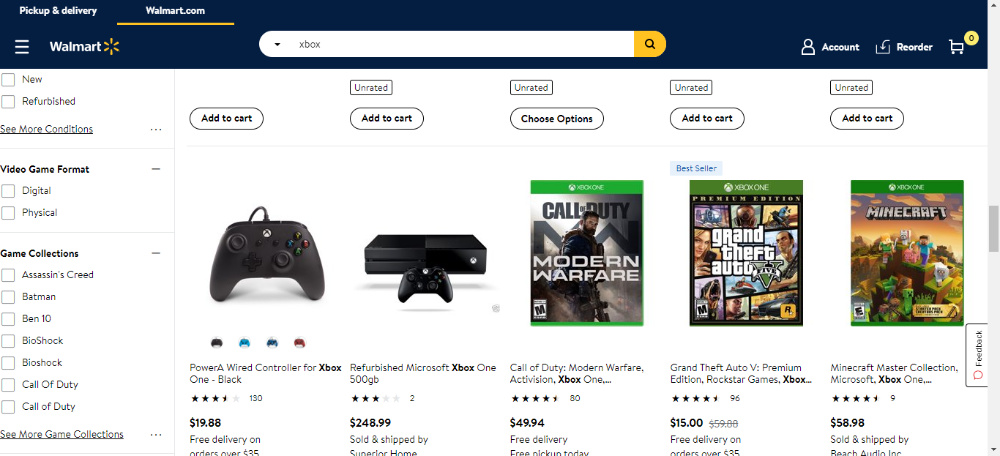A user is browsing the Walmart desktop website and has entered 'Xbox' into the search bar at the top of the page. The navigation bar is navy blue, and it includes the search bar, which is white with a yellow search button featuring a magnifying glass icon. The cart icon shows a zero, indicating that there are currently no items in the cart. Links for account access and reordering are also visible. 

As the user scrolls down halfway through the search results, they encounter several Xbox-related products: a PowerA wired controller for Xbox One priced at $20, a refurbished 500GB Xbox One console with Call of Duty: Modern Warfare for $250, the game Call of Duty: Modern Warfare for $50, Grand Theft Auto V (GTA V) at a notably discounted price of $15 (down from its original $60), and the Minecraft Master Collection for $59. Each item has an 'Add to Cart' button next to it, enabling easy purchase directly from the search results.